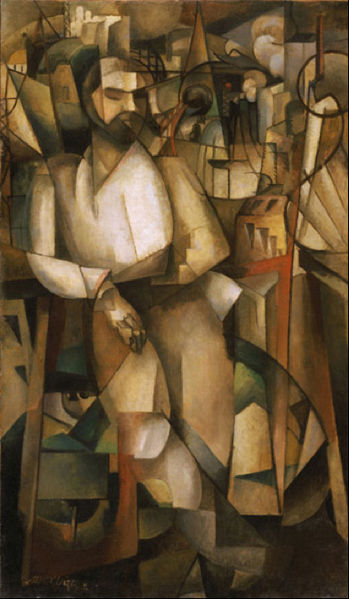This painting, rendered in a Cubist style, depicts a man standing in the center, characterized by a muted palette of browns, beiges, and occasional hints of orange and green. The man's head, clearly visible with a beard and upwards-slanting eyes, appears bald. He is dressed in a white vest and tan long pants, with his right leg crossed over his left and his right hand extended down to the lower part of his right leg. He leans to his right against a complex, overlapping arrangement of geometric shapes, including cubes, triangles, circles, rectangles, and squares. These shapes, blending and blurring into one another, form an intricate, multi-dimensional background. The composition includes the illusion of additional faces formed by the interlocking outlines of various shapes. The innovative use of geometric forms and muted colors creates a layered, modern, and dynamic visual experience.